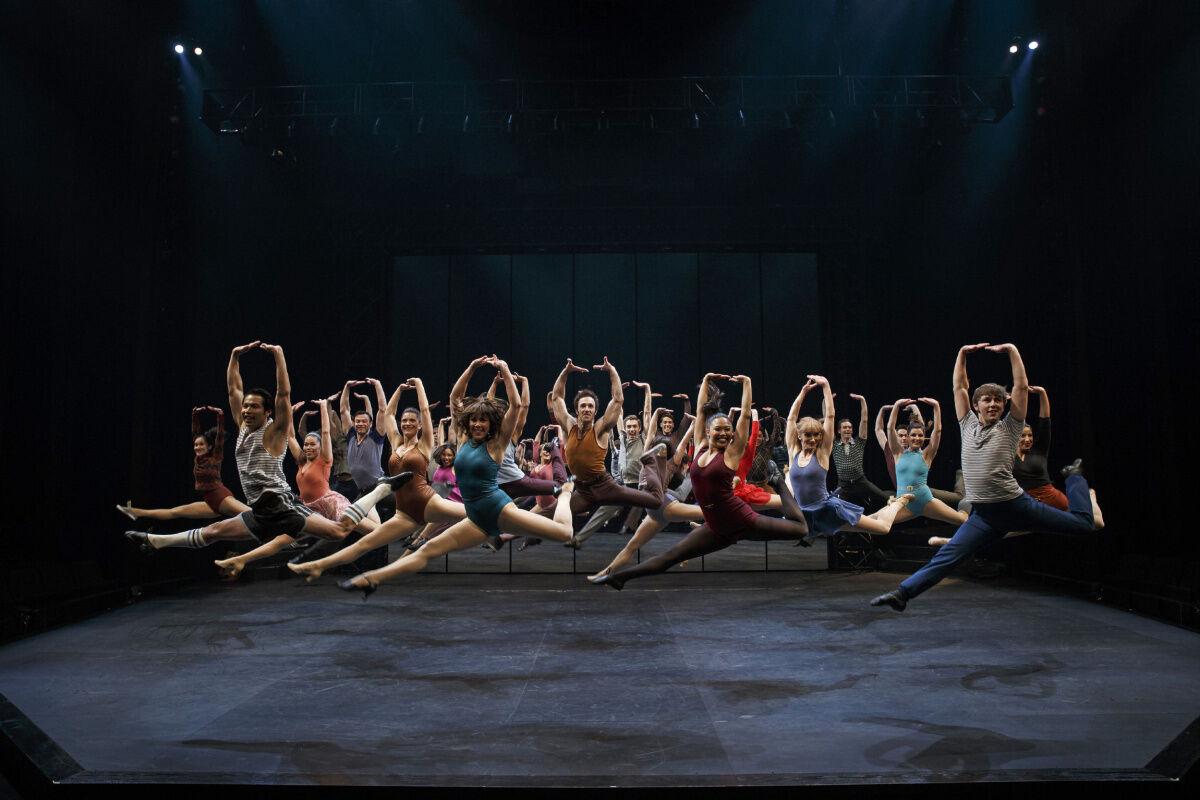The photograph captures a vibrant ensemble of over 20 dancers, both male and female, performing a perfectly synchronized jump on a dark stage. Each dancer exhibits an impressive split jump with one leg stretched forward and the other leg bent backward, toes pointed towards their heads. Their arms are elegantly extended above their heads with fingers touching or palms facing the ceiling. The dancers, dressed in a mix of skirts, tank tops, shorts, and various colors, display a diverse range of ethnicities. Some wear shoes while others appear to be barefoot or in minimal footwear. The stage itself is enveloped in black, accentuating the dancers' brightly colored attire and the dramatic pose. Four high spotlights illuminate them from above, casting shadows on the black stage floor and creating a striking visual contrast that highlights the grace and coordination of their jump.